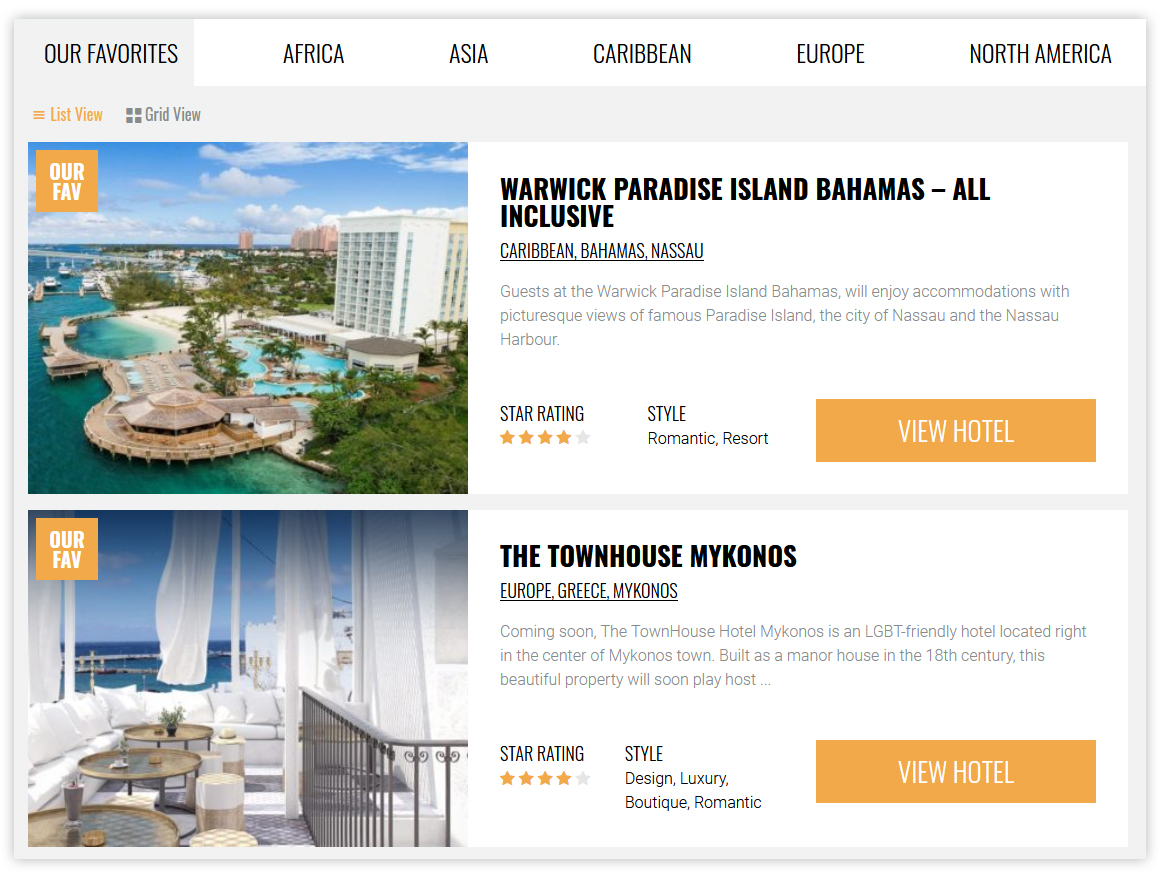The image showcases a selection of top travel destinations around the globe, prominently featuring favorites such as Africa, Asia, the Caribbean, Europe, and North America, highlighted in a white bar at the top of the image. Below are options to view the list in an orange button or switch to a grid view in a gray button.

The first featured destination is the Warwick Paradise Island in the Bahamas. This stunning aerial shot captures the resort set against the backdrop of crystal-clear blue waters adorned with palm trees and boats. The resort itself showcases a pristine white building, complemented by a luxurious swimming pool. Beyond the resort, tall buildings of Nassau are visible. Descriptive text highlights that guests at Warwick Paradise Island, Bahamas, will enjoy accommodations with picturesque views of the famous Paradise Island, the city of Nassau, and the Nassau Harbor. The resort has a four-star rating and is styled as a Romantic Resort. There is an orange "View Hotel" button for more details.

Beneath this, another highlighted destination is the Townhouse Mykonos, located in the heart of Mykonos Town, Greece, Europe. "Our Favorite" is marked in an orange box within the image. The description mentions that this LGBT-friendly hotel, originally an 18th-century manor, is currently under development. It's expected to provide a luxurious stay with a four-star rating and a design that merges luxury, boutique, and romantic styles. Like the Warwick Paradise, there is also an orange "View Hotel" button available for further information.